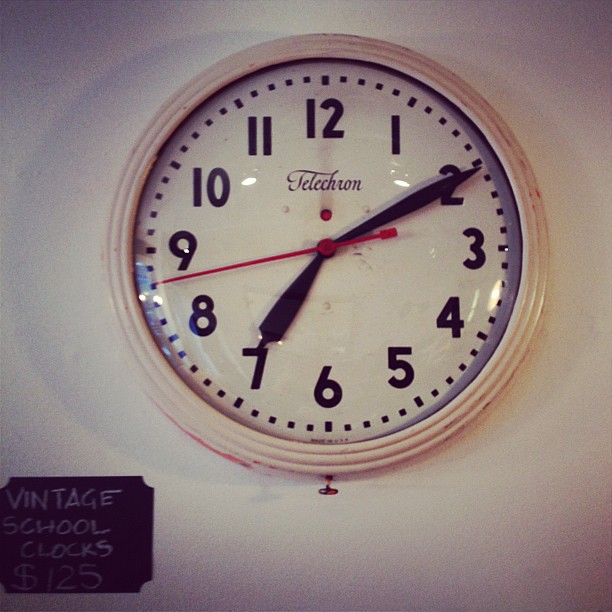This low-quality, dark photograph depicts a vintage Telechron school clock, reminiscent of those found above blackboards in 1970s classrooms. The clock features a circular white face with plain black numerals and black tick marks denoting the minutes. It has black hour and minute hands, along with a red second hand currently positioned between the 8 and 9. The clock is encased in a beige outer frame with three distinct levels. Centered on the clock face is a red dot and the brand name "Telechron" written in cursive script. At the bottom left corner of the image, a black chalkboard-style price tag displays "vintage school clocks $125" in white chalk-like handwriting. The clock casts a shadow on the wall behind it, and the time shown is 7:10. The overall appearance of the clock is dingy and dirty, matching the aged, nostalgic feel of the item.